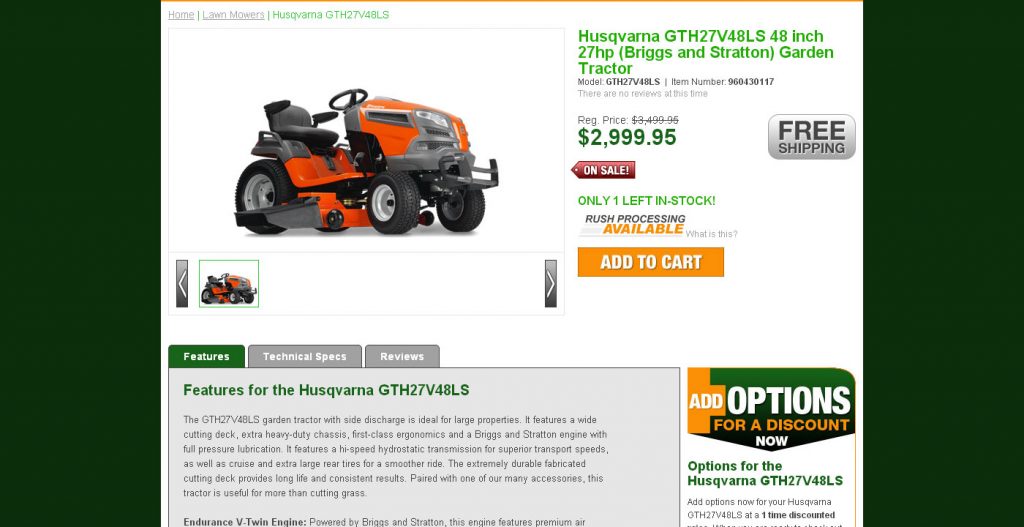The image features a detailed promotional layout for a Husqvarna garden tractor, showcasing a riding lawnmower model in vivid detail. The central section of the image is set against a white background, framed by dark green borders on the left and right sides, with a thin orange line accentuating the top of the white background.

In the middle of this layout, there's a prominent image of an orange and gray Husqvarna riding lawnmower. To the right of this image, green text displays the model and specifications: "Husqvarna GTH27V48LS, 48 inch, 27 HP (Briggs & Stratton)." Further below, black text states the model number once more: "Model GTH27V48LS."

Directly underneath this model information, the price is highlighted in dark green text: "$2,999.95." Enhancing the urgency of the offer, a red banner immediately below the price announces "On Sale." Adjacent to this, a gray box with black text offers "Free Shipping."

Adding to the call to action, green text informs potential buyers that there is "Only one left in stock." Beneath this, black and orange text alerts customers to the availability of "Rush Processing Available." Finally, at the bottom of the promotional layout, an orange button with white text encourages immediate purchase with "Add to Cart."